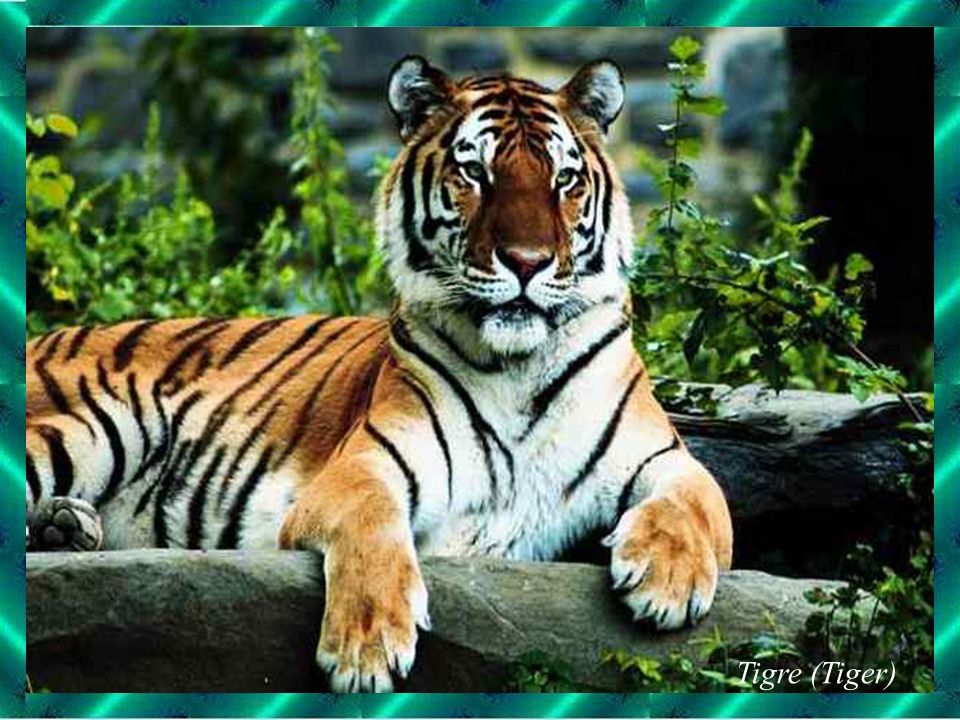This detailed photograph centers on a stunning Siberian tiger, depicted in its natural forest habitat. The tiger, showcasing its distinctive bright orange fur with bold black stripes, contrasts sharply with its white underbelly. With alert green eyes and short ears, the tiger rests majestically atop a fallen log, gazing left towards the edge of the frame, creating a sense of vigilant calm. Surrounding the tiger is a lush green foliage, featuring trees, bushes, and twigs, some in sharp focus while others fade into a blurred background, enhancing the depth and authenticity of the forest environment. The image itself is bordered by a greenish, iridescent frame, adding a unique touch to the scene. At the bottom of the picture, the word "tigre" is prominently displayed with "tiger" in parentheses, identifying the magnificent creature. The color palette of the photograph includes vivid shades of orange, black, white, green, brown, gray, and beige, capturing the essence of the wild. The photo is a square shot, reinforcing its classic aesthetic appeal as a natural wildlife portrait.